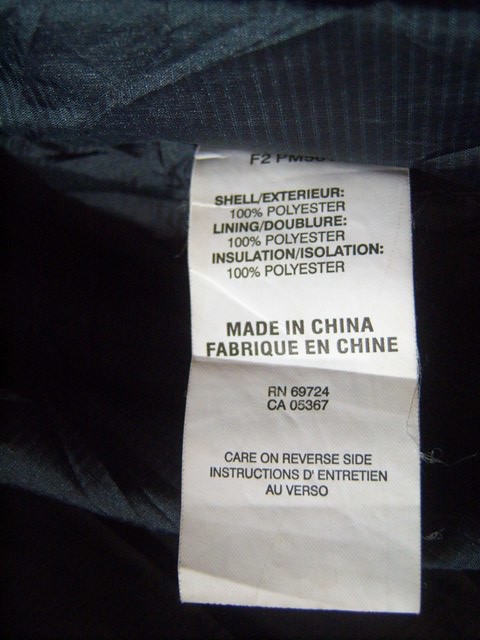The image is a close-up of a white rectangular tag attached to a dark background, possibly a pillow, sweatshirt, or sweater. The tag is folded in the middle, creating a crease from the left center to the right center. The tag has black text which starts at the top, partially cut off, reading "F2" followed by an unclear portion. Below this, the tag alternates between English and French, stating: "Shell exterior 100% polyester," "Lining doublure 100% polyester," and "Insulation/Isolation 100% polyester." Further down, the text reads "Made in China" and "Fabrique en Chine." The tag also includes smaller print: "RN-69724" and "CA-05367." At the bottom, it instructs to "Care on reverse side" and provides the French translation: "Instructions d'entretien au verso." The tag appears to be in good condition with clear, legible text.